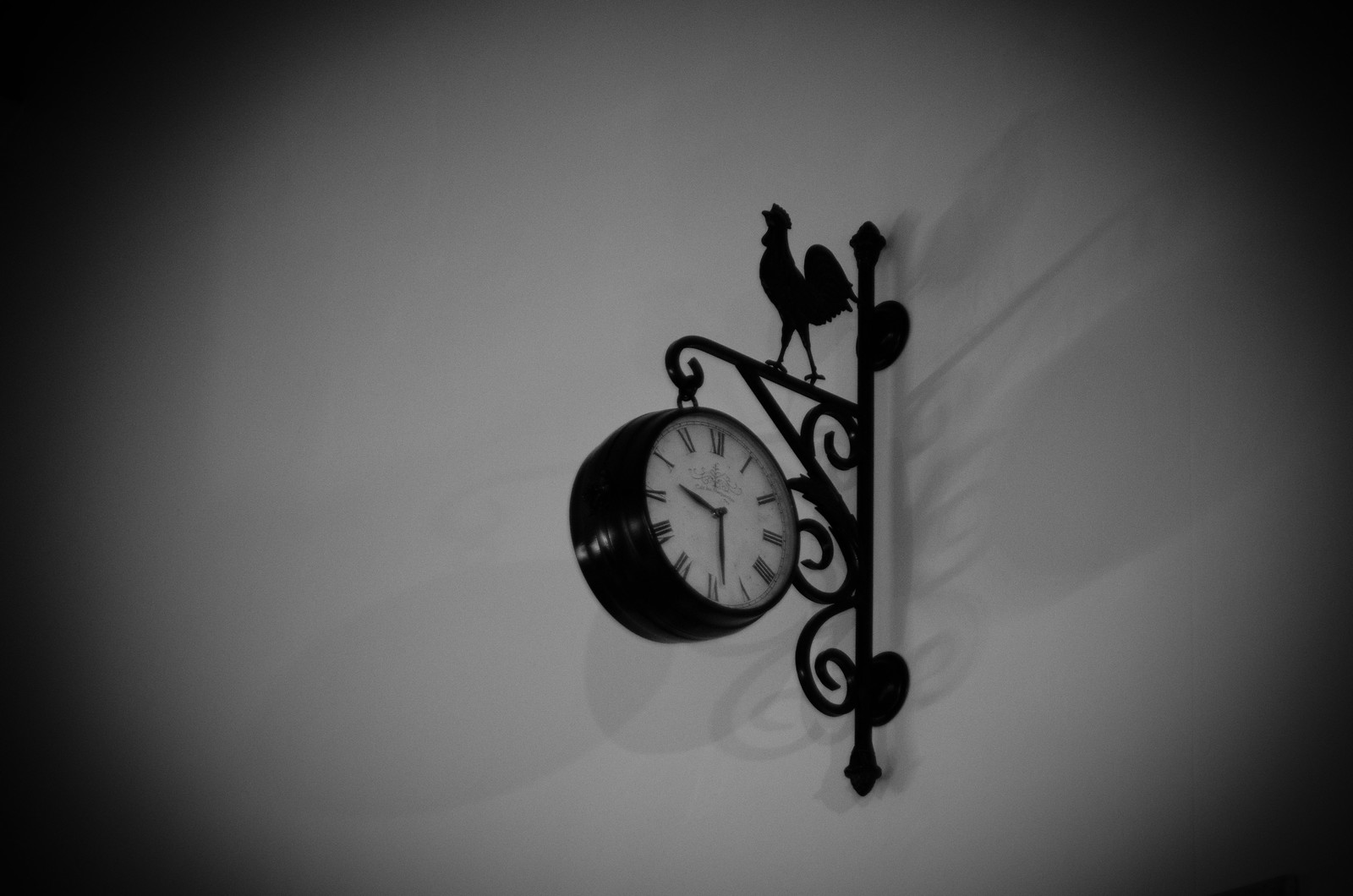This black-and-white landscape photograph captures a beautifully designed, large wall-mounted clock, taken from a low angle looking upward, suggesting its considerable size. The clock, featuring black Roman numerals on a white face and a clear hour and minute hand, hangs from an elaborately decorated wrought iron bracket. The bracket, attached to a white wall at two points, extends outward, culminating in a silhouette of a cockerel perched above. The clock is encased in a thick, black frame and shows the time as either half past nine or 10:30. The photo's edges are enveloped in darkness, creating an oval vignette that focuses attention on the clock, with shadows cast on both sides indicating a central light source.